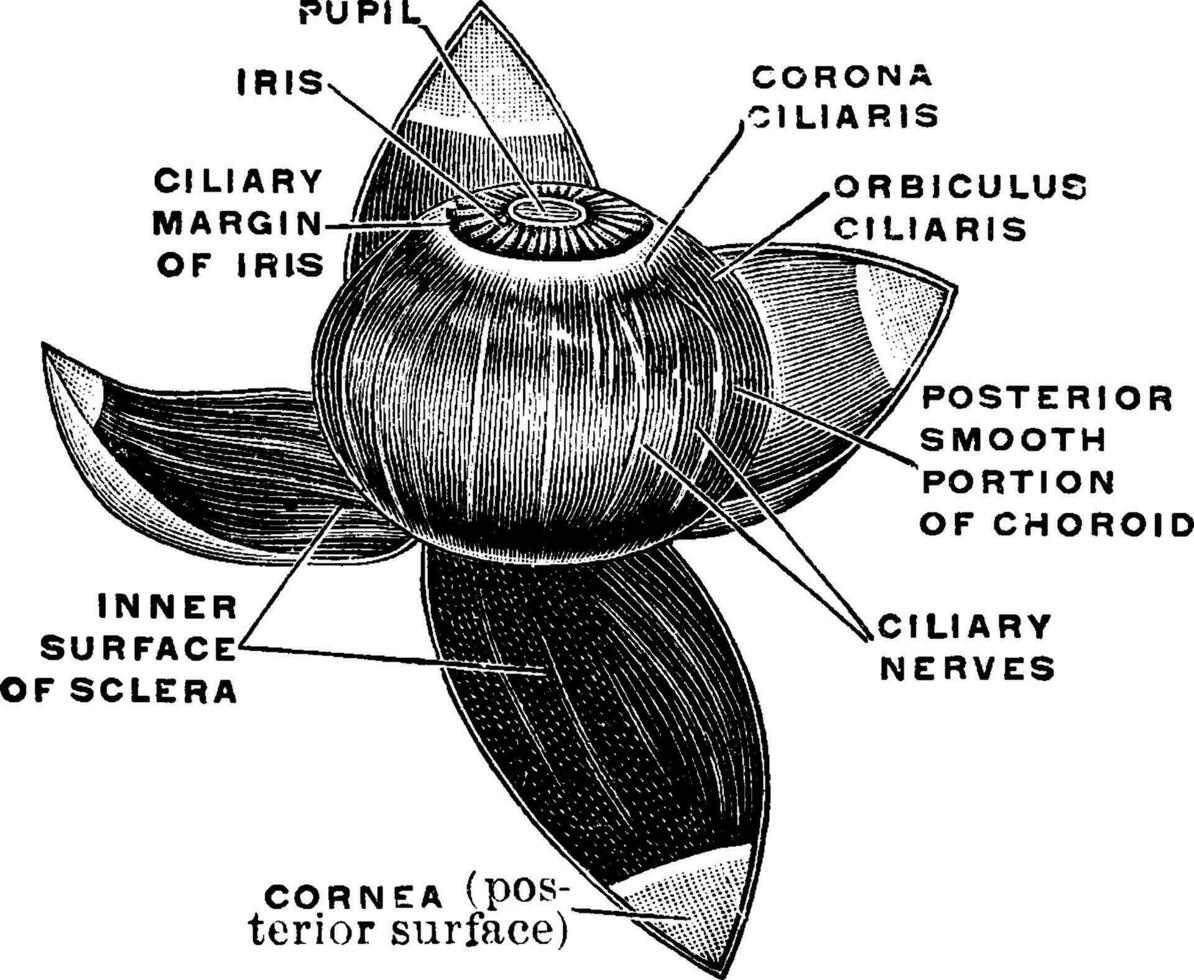This is a detailed black and white hand-drawn diagram of the human eye, created with fine black pen or pencil. The central focus of the image is a full, round eye orb featuring the pupil and iris. Surrounding the eye, there are four petal-like structures extending outward, giving an almost floral appearance. These structures contribute to the intricate design by acting as cutaways, revealing detailed anatomical features of the eye. The meticulous drawing is densely populated with black lines adding depth and detail to the various components, which are clearly labeled. The labels, positioned in a clockwise manner, include: pupil, iris, ciliary margin of iris, corona ciliaris, orbiculus ciliaris, posterior smooth portion of choroid, ciliary nerves, inner surface of sclera, and cornea (posterior surface). Each label is connected by a line to its respective part, making the diagram not only artistically striking but also highly informative. The entire image is devoid of any color, set against a plain white background with text in black, maintaining a consistent and clean visual theme.